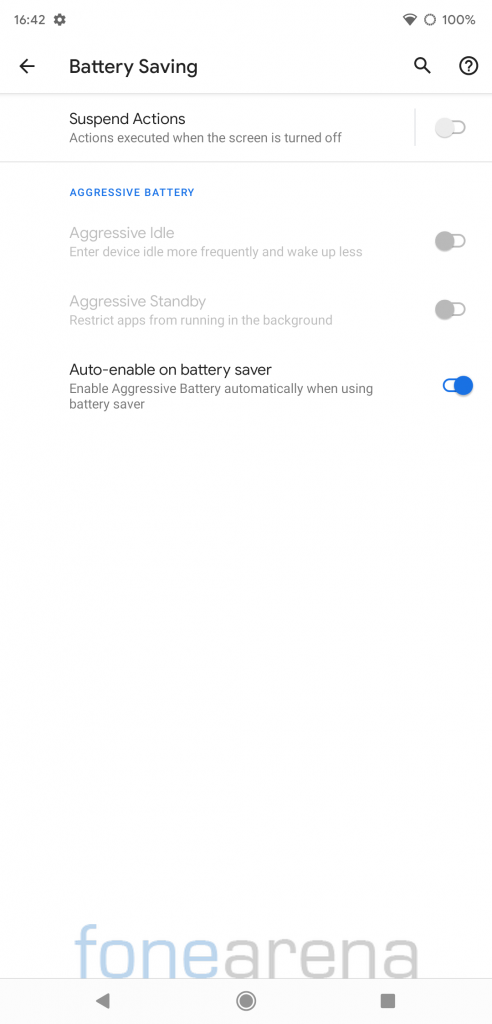This image is a screenshot taken from a mobile device, featuring a white background. At the top, there are dark grey icons indicating the time, a settings cog, Wi-Fi connection, and battery status. At the bottom, grey navigational buttons are visible, including a backward-facing triangle, a circle, and a square icon. Just above these buttons, there is a watermark with blue and grey text that reads "fone arena," with 'fone' spelled using an 'F'. The screenshot showcases a settings menu titled "Battery Savings." Within this menu, there are several toggle options including "Suspend Actions," "Aggressive Idle," "Aggressive Standby" (all of which are currently deselected), and "Auto Enable on Battery Saver" (which is selected).